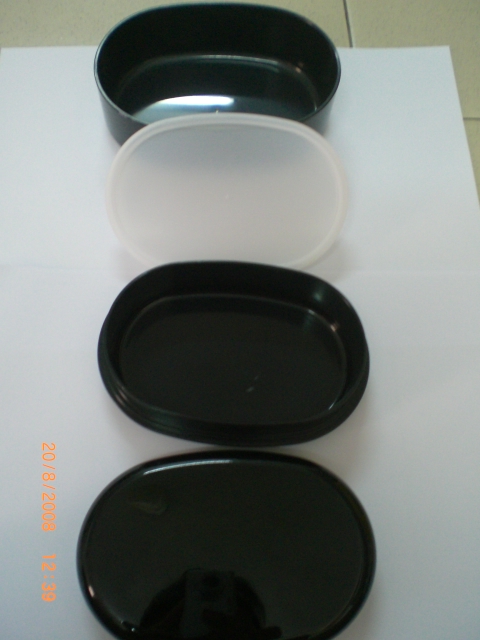This is a detailed, above-angle color photograph taken on August 20, 2008, at 12:39 PM, capturing three shiny black plastic containers of varying shapes and sizes laid out on a white piece of paper. The containers are positioned on a beige-tiled floor, where the grouting is visible. At the top of the image, there is a deep black oval container with an opaque white lid leaning against it. Below, two shallower black oblong containers are laying flat. The photograph displays the reflection of the photographer's head and phone within the shiny surface of the containers. The date "20-8-2008" is noted in orange font in the bottom left corner of the image.